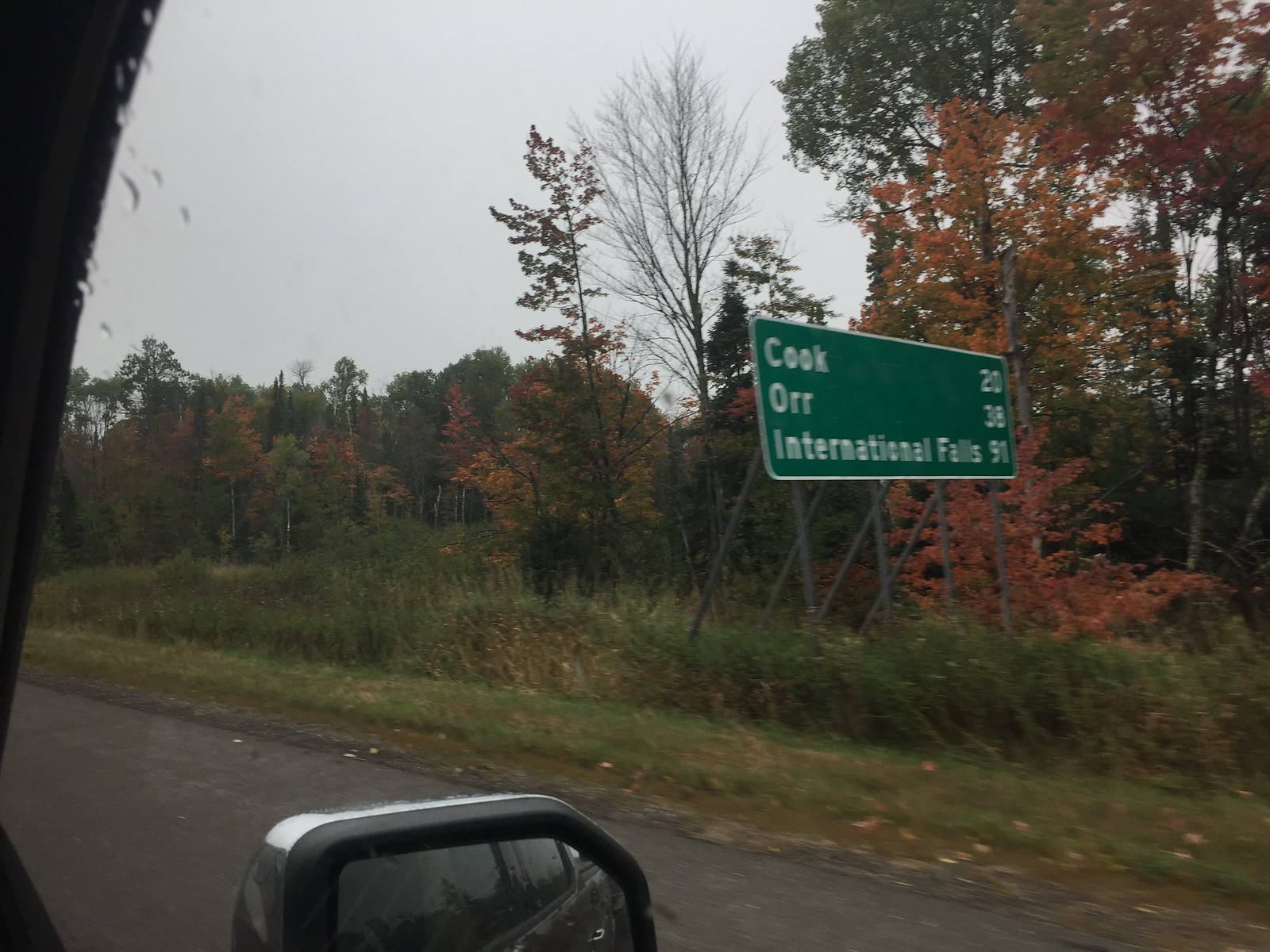In this horizontally oriented photograph, taken from the side window of a vehicle on a somewhat cloudy day, we capture the essence of an autumn journey. The side view mirror and a glimpse of the car's interior frame the scene, providing context. Outside, a picturesque autumn landscape unfolds, with trees displaying a vibrant array of golden, red, and green foliage lining the paved road. A green road sign with white lettering stands prominently, reading "Cook 20 miles" and "International Falls 91 miles." The roadside is peppered with fallen leaves scattered across patches of dirt and grass, punctuating the seasonal ambiance of the drive.